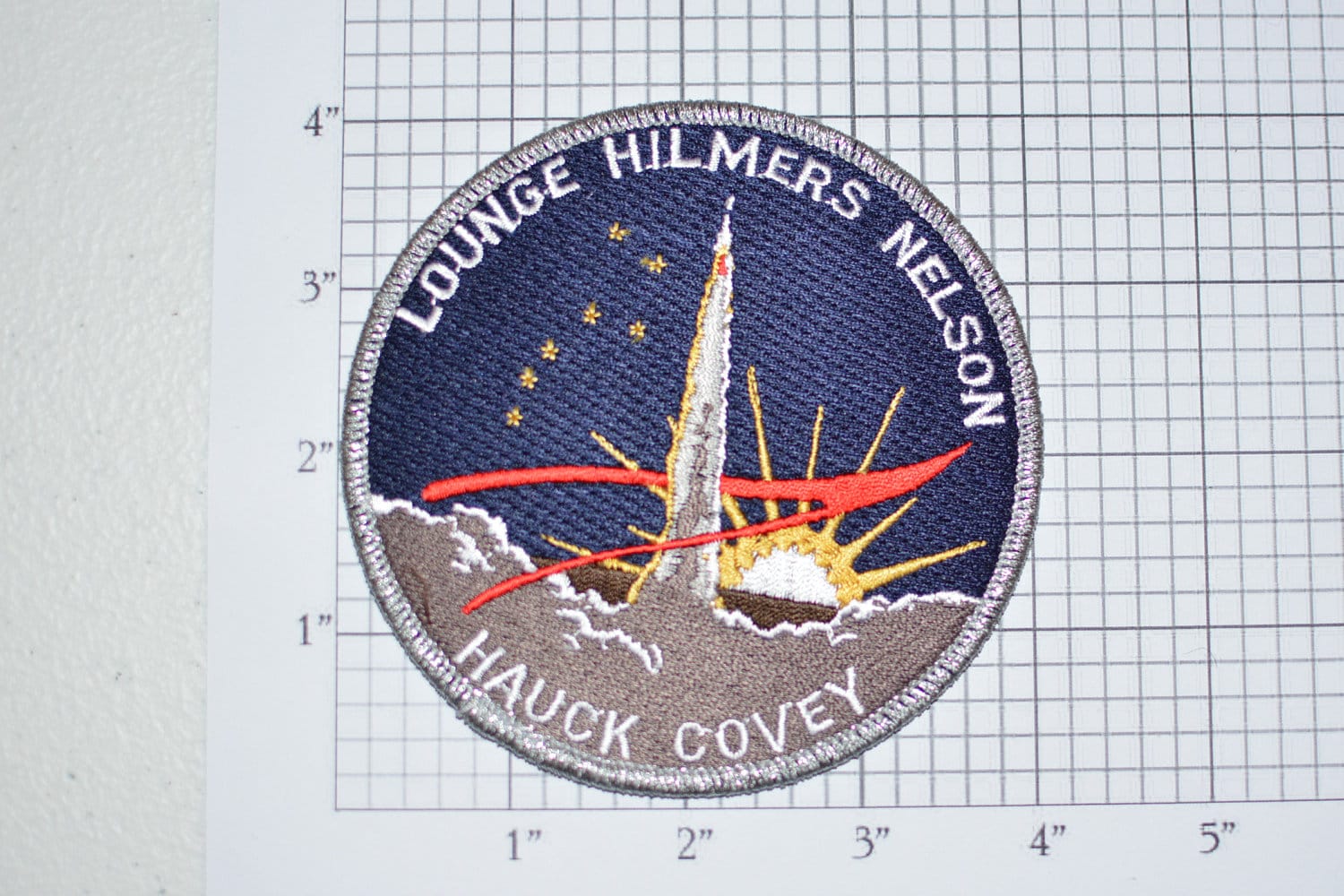The image depicts a round, sew-on fabric badge, measuring approximately 4 by 4 inches, displayed on graphing paper marked with one-inch increments along both axes. The central design features a space rocket launching amidst a billow of grey clouds, with a half-sunburst set against the upper background, evoking the sensation of a dawn skyline. The badge carries the text "Lounge Hilmers Nelson" prominently at the top, with the phrase "Hauk Covey" at the bottom, suggesting possible affiliations or names. The color scheme includes shades of blue, gold, white, and red, further accentuating the celestial and dynamic theme of the imagery.